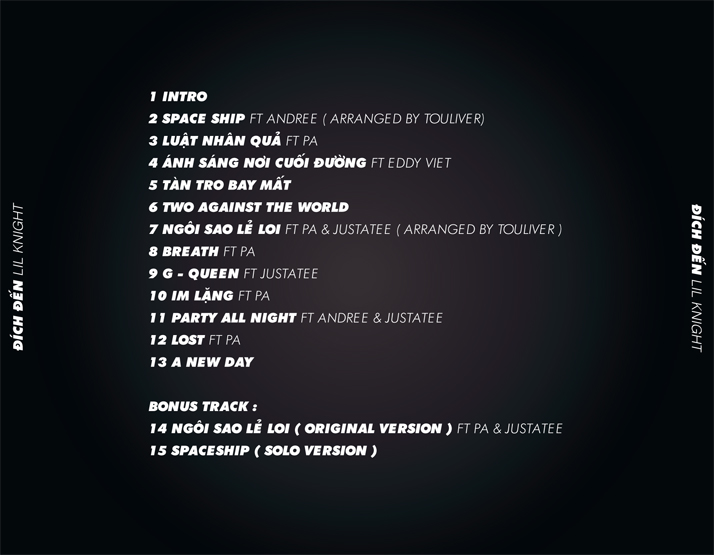The image features the back cover of a music album with a black background and white text. The title "Dikden Little Night" is prominently displayed on both the left and right sides. In the middle of the image, a detailed numbered list of songs is presented, including both English and foreign language titles, likely Vietnamese:

1. Intro
2. Spaceship featuring André, arranged by Tuliver
3. Roots featuring P.A.
4. An Sang Noi Khoi Duong, featuring Eddie Viet
5. Tanstru Baymat
6. Two Against the World
7. [Title in an unidentifiable language]
8. Breath featuring P.A.
9. G / Queen featuring Justa T
10. [Title in an unidentifiable language]
11. Party All Night featuring André and Justa T
12. Lost featuring P.A.
13. A New Day
14. Ngiyo Sai original version, featuring P.A. and Justa T (Bonus Track)
15. Spaceship (Solo Version)

The text provides a mix of song titles and featured artists, emphasizing the multicultural aspect of the album.